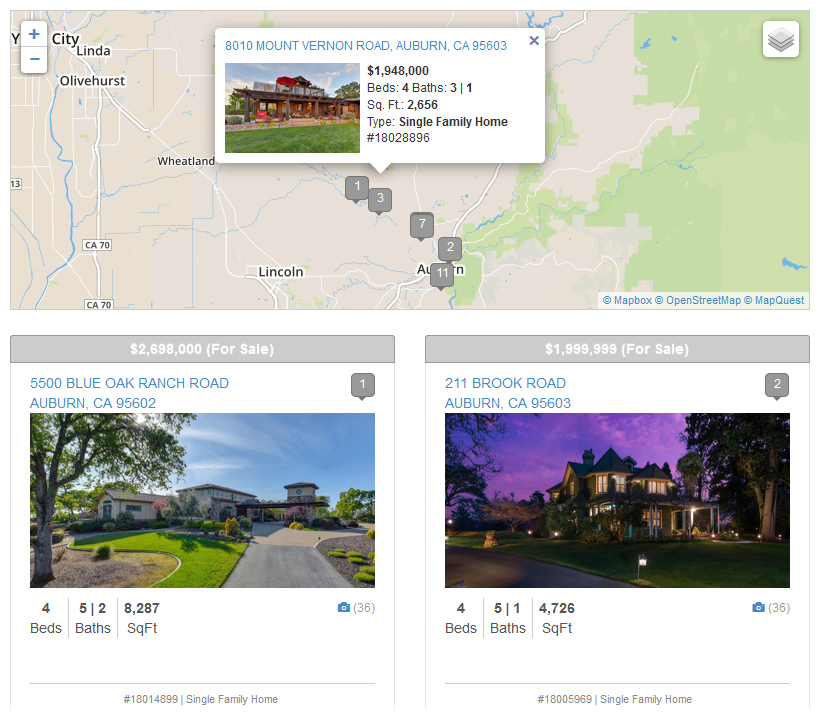Here's a more refined and detailed caption for the described image:

---

The image is a screenshot of a real estate website interface for buying and selling homes. The background is predominantly white, with a large map taking up the top portion of the page. The map is rendered in shades of gray, with city names written in black, delineated roads, and patches of green representing foliage, particularly on the right-hand side.

In the middle of the map, several small gray boxes with white numbers (1, 3, 7, 2, and 11) are displayed. A highlighted property, indicated by the number 3, has a white pop-up box above it. This box is headed with the address "8010 MOUNT VERNON ROAD, AUBURN, CA 95603" in blue, uppercase letters. 

To the left of the address, there is a thumbnail image of a single-story, brown brick house with green grass, a clear sky, and some green trees, suggesting the photograph was taken during the spring or summer months. To the right of the image, the property price is listed as "$1,948,000." Below this, in gray font, the details "Beds: 4, Baths: 3, Sq Ft: 2,656" are provided, followed by the property type, "Single Family Home," in bold black text.

The remainder of the page continues with a white background and includes two elongated gray buttons below the primary property listing. The button on the left reads "$2,698,000 (For Sale)" in white text, while the button on the right displays "$1,999,999 (For Sale)." The page also lists other addresses and comparable large mansion-type houses, along with their respective bed, bath, and square footage details.

---